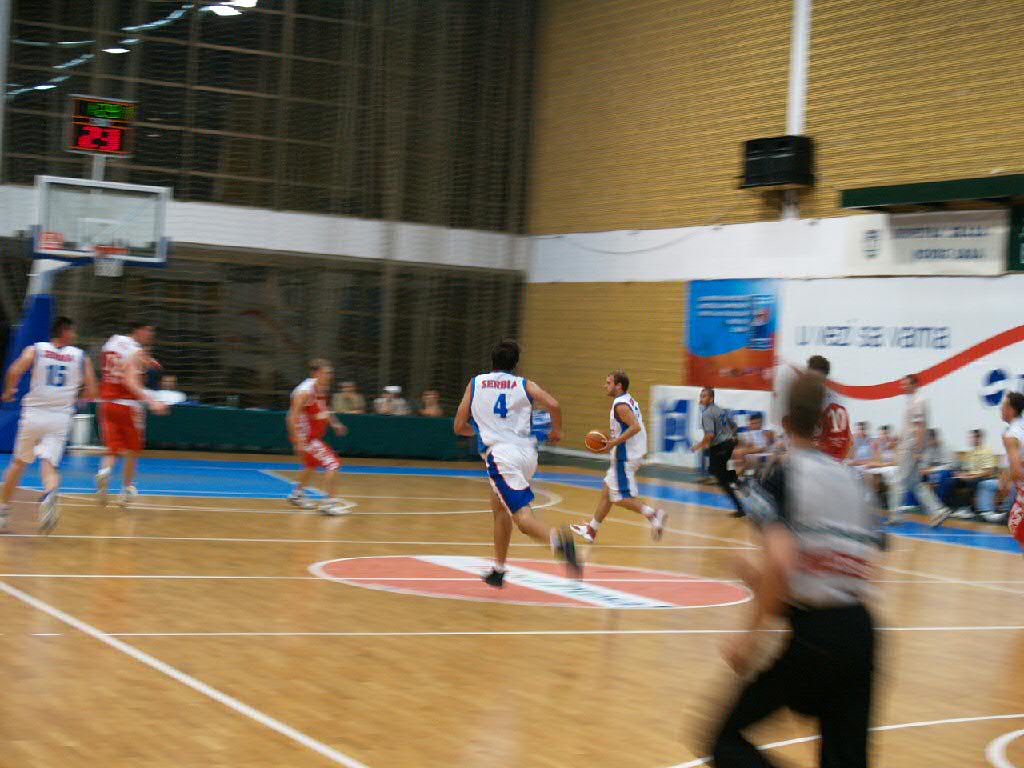The image captures an intense moment from a high-energy basketball game, taken from a corner angle that spans diagonally across the court. The backdrop features a brick wall on the right side and a series of windows divided by bronze iron on the left. A basketball hoop is positioned high on the left side, with a scoreboard displaying a score of either 23 or 29 in red above it.

In the foreground of the left corner, two players are visible: one sporting a white and blue uniform, and the other clad in red and white. Just inside the three-point line stands another player in a red and white uniform, with a fair complexion. Dominating the central circle is a black player wearing a white and blue uniform prominently displaying the number four. Nearby, to the right, is a shorter white player, also in a white uniform with a blue stripe, who is actively dribbling the basketball.

A referee is positioned closely on the right side of the image, though he appears slightly blurry. Another referee can be seen running along the right edge of the frame. In the background, along the sideline, a cluster of players or coaches are seated on benches, attentively observing the proceedings of the game.